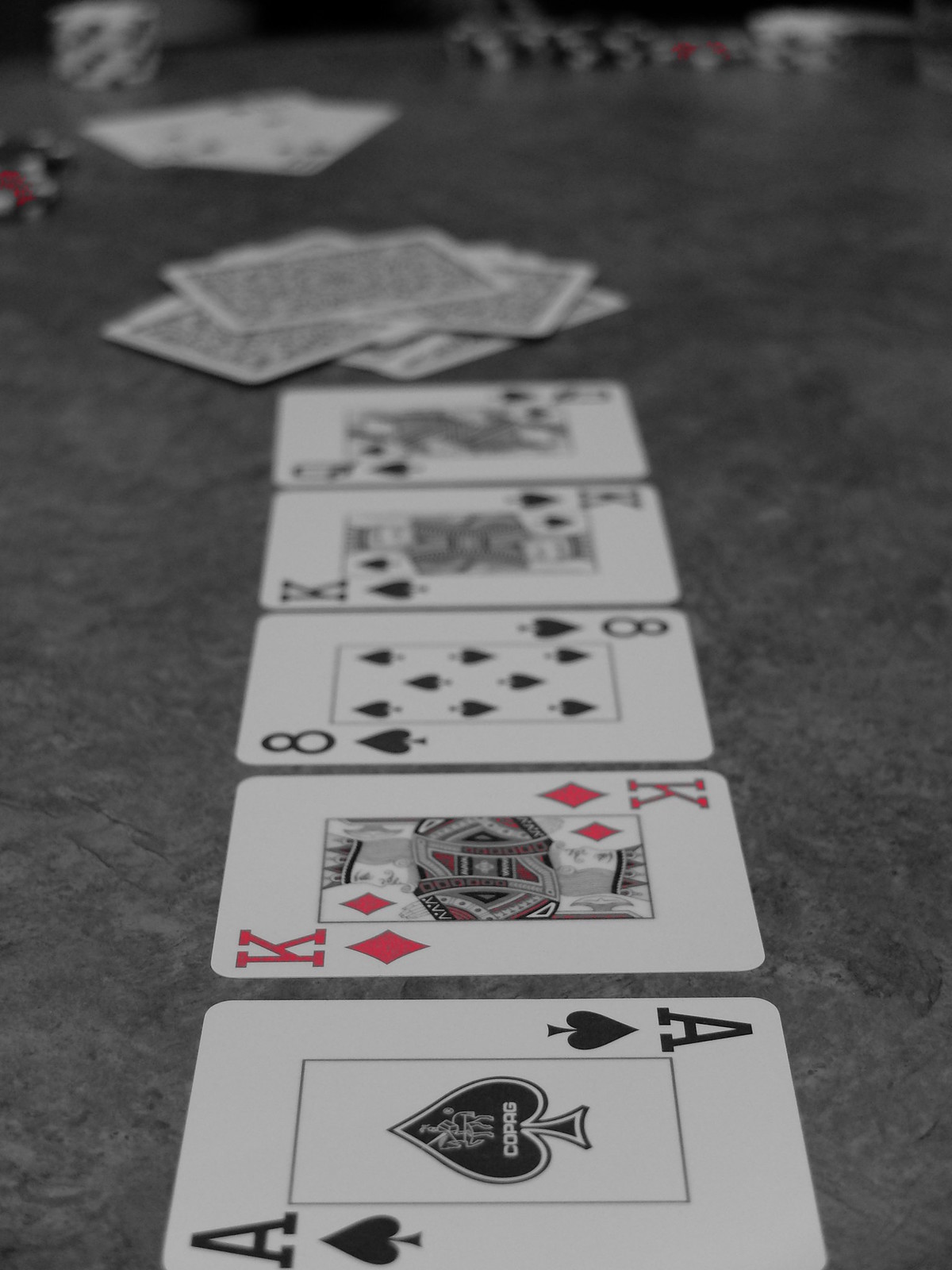The photograph features a neatly arranged series of playing cards displayed on a sleek, gray marble table, exuding elegance and professionalism with its mottled white and darker gray patterns. The image is vertically oriented, with the focal point being the cards in the foreground. At the top left corner, a blurry stack of white and gray poker chips can be seen, suggesting a poker game context. Additional poker chips, including black, white, and a few with a red hue, are scattered around the top right corner. Some stacked playing cards and red, black, and white chips are also visible on the left side of the image, although these elements are slightly out of focus to emphasize the cards in front.

In the foreground, a clear arrangement of six playing cards is laid out horizontally, from the farthest to the closest: a Queen of Clubs, King of Spades, another King of Spades, an Eight of Spades, a King of Diamonds, and an Ace of Diamonds. Two face-up cards with black suits are positioned near the top left, hinting at ongoing gameplay. Additionally, a small booklet lies closer to the viewer. A pile of face-down cards with a white border and a spotted gray pattern on their backs completes the composition, adding to the sophisticated ambiance of this poker setting.